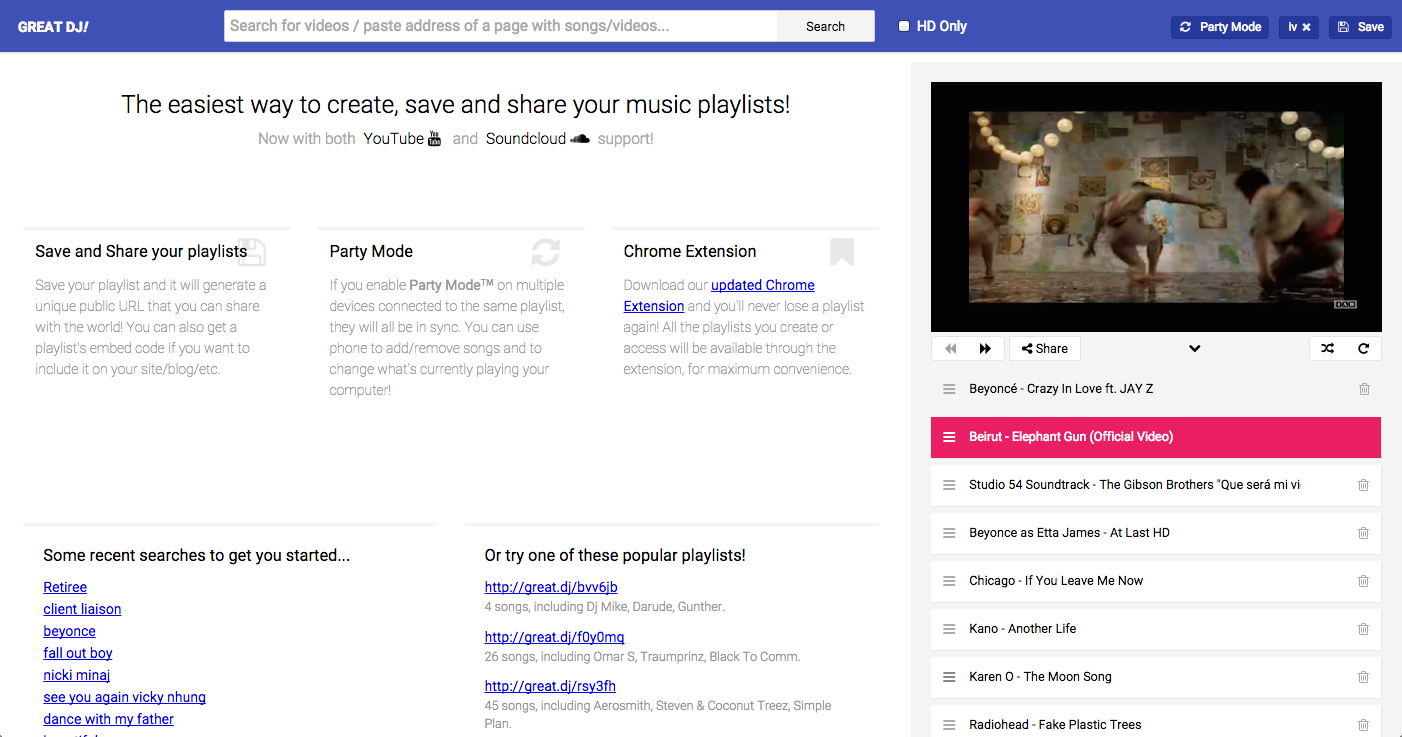The displayed image is a webpage with a well-structured design. At the top, there is a medium-dark blue banner. On the top left corner, prominently written in all capital letters, is the phrase "GREAT DJ!". Adjacent to this on the right, there is a white search bar with the placeholder text: "search videos/paste address of a page with songs/videos...". Next to the search bar, there is a light gray search button labeled with the word "Search" in capitalized black text.

Moving further to the right within the blue banner, there's a small box labeled "HD ONLY," both words emphasizing the high-definition feature with capital letters. Along the right side of the banner, there are multiple option squares. The first square features white text reading "Party Mode" followed by "IVX" also in white text. Another option available in this area is a save feature, denoted simply with "Save" in capitalized white text.

Below the banner, the page transitions into a white background. Centered on the left side of this section, there is a large, clear message that reads: "The easiest way to create, save, and share your music playlist!" This is followed by a notification of extended support: "Now with both YouTube and SoundCloud support." Below this informative text, users are encouraged to "Save and share your playlist" and mentioned is an additional "Party Mode Chrome Extension".

At the bottom of the central area, a section titled "Some recent searches to get you started" provides hyperlinked options for quick access. Alongside this, the prompt "Or try one of these popular playlists" followed by web addresses invites users to explore curated content.

On the right side of the page, a graphic illustration is displayed, contributing to the website's engaging visual elements. Below this graphic, different lists and songs are mentioned, enhancing the appeal for users seeking various musical options.